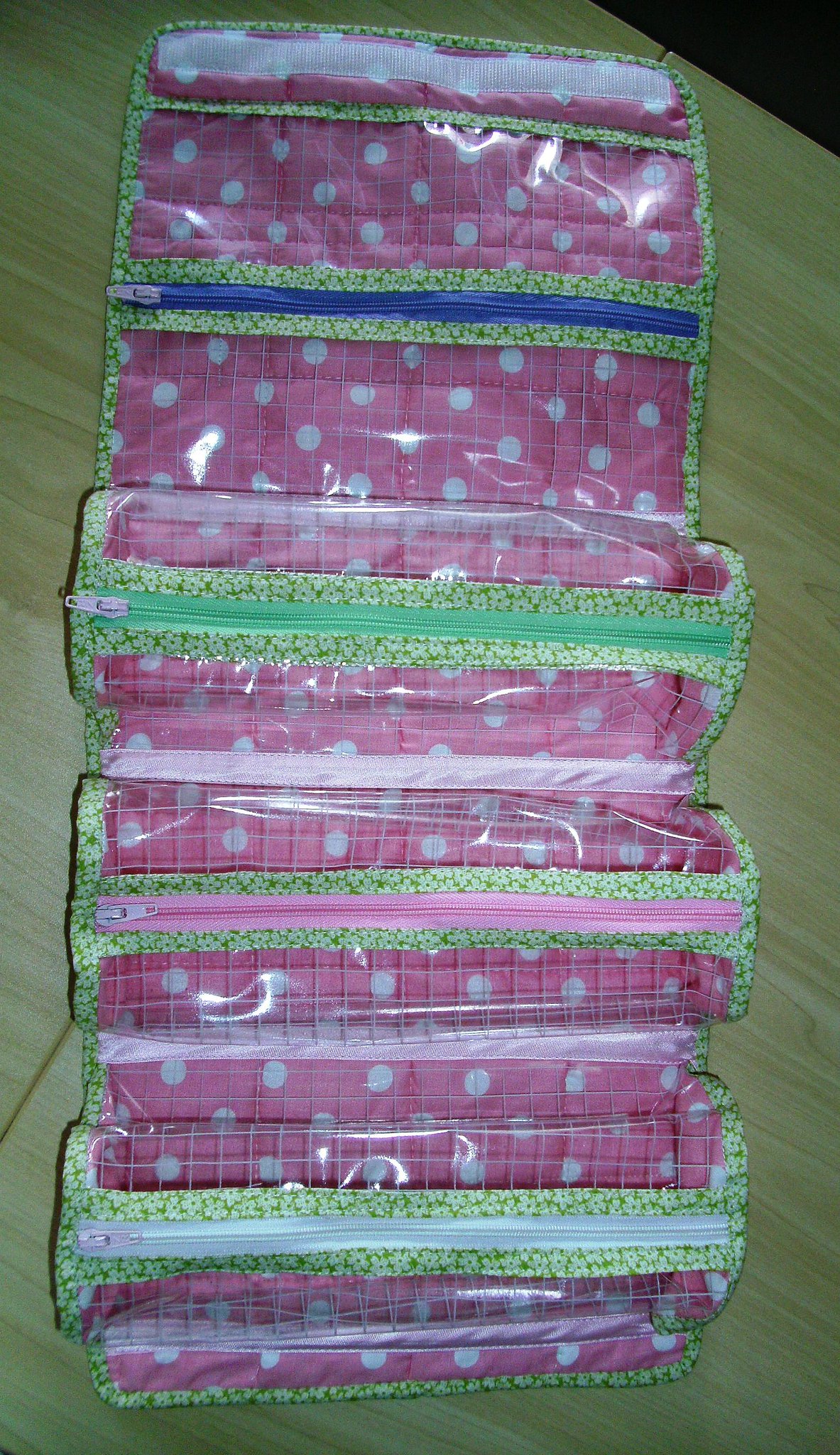This is a photorealistic image of four plastic zippered pouches, likely pencil cases or travel accessories for storing small items. They are arranged on a white-painted wooden table, viewed from above, with three of the pouches standing up and one lying down. Each pouch features a dark pink background adorned with white polka dots and different colored zippers—one blue, one green, one pink, and one white—each zipper has a white fastener. The pouches also have a Velcro closure and appear to be padded or made of quilted fabric for extra durability. There is green trim around the sides of the pouches, accentuating their design. The lighting in the image is dim, suggesting it was taken in an unlit room.